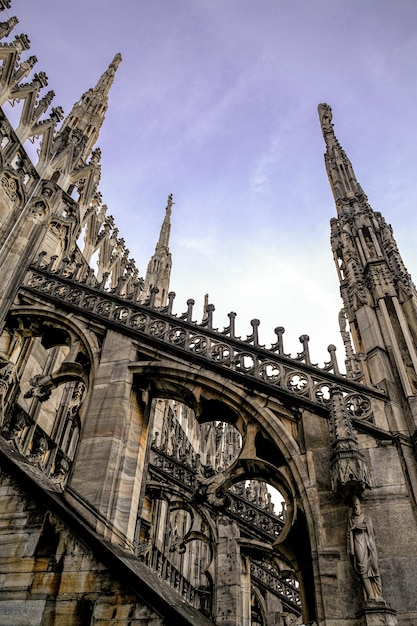This vertically oriented photograph captures a stunning Gothic cathedral against a clear blue sky dotted with white clouds. Taken from a low angle, the image showcases the towering spires and intricate stonework that define the architectural marvel. The stone structure, adorned with ornate designs and spikes, exhibits the craftsmanship of a bygone era. Prominent features include a flying buttress and what appears to be an archway or stairway ascending across the photograph from left to right. The stone, predominantly gray with occasional stripes of red, adds to the stark, historical allure of the cathedral, making it a captivating sight against the vivid sky.